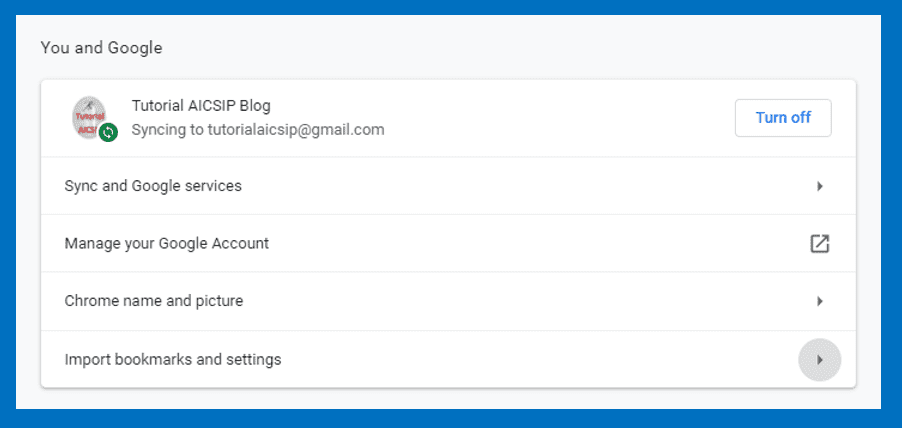This image captures a structured interface titled "You and Google" positioned at the top left. Directly beneath this heading are five distinct sections, each serving a unique function related to Google account management. 

The first section, labeled "tutorial AICSIP blog syncing to tutorial AICSIP at gmail.com", features a gray circle with red text reading "tutorial," accompanied by a green circle adjacent to it. To the far right of this section is the option to "Turn off" displayed in blue text.

Following this are four neatly arranged sections from top to bottom:

1. **Sync and Google Services** - Marked with a small arrow to the right.
2. **Manage your Account** - Connected to the "Manage your Google account" option featuring a share icon.
3. **Chrome Name and Picture** - Highlighted with a small arrow.
4. **Import Bookmarks and Settings** - Distinguished by a gray circle and arrow.

The interface delineates sections with a white background, while the topmost area has a gray backdrop. Surrounding the entire frame of the image is a soothing blue background, providing visual separation from the main content.